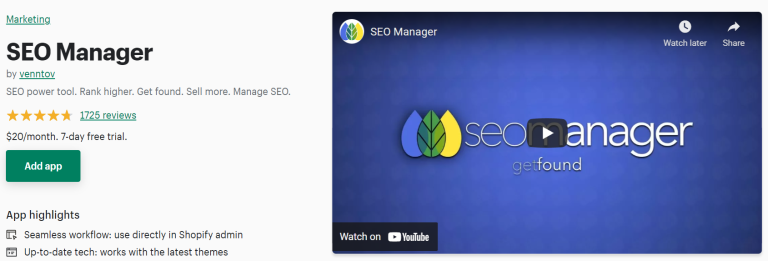**Detailed Caption for the Marketing Website Image:**

The image depicts a detailed interface of a marketing website, specifically focusing on an SEO management application. On the left-hand side, within a white square, "Marketing" is highlighted in blue at the top left corner. Directly below is the label "SEO Manager" in bold black text. Further down, the word "Buy" appears in gray, followed by the term "VENNTOV," which is highlighted and underlined. Moving down, "SEO Power Tool, rank higher, get found, sell more, manage SEO" is displayed in gray text.

Next, a section with five highlighted stars is shown, indicating a rating. To the right of the stars, the text "1,725 reviews" is highlighted in green. Continuing downward, "$20/month," "7-day free trial" is stated in black. Below this, a green button with the text "Add App" in white is present.

Further down the left side, there’s a heading "App Highlights" in black. Underneath, a small square with a right-facing arrow is present, followed by "Seamless Workflow, used directly in Shopify Admin" in dark gray. Another small square is present below, next to which "Up-to-Date Tech, works with the latest themes" is written in gray text.

To the right of this section, a blue rectangular area appears to be a pop-up resembling a YouTube play screen. The background is entirely blue, featuring a circle with three leaves (one blue, one green, and one yellow) in the top left corner. To the right of the circle, "SEO Manager" is written in gray. Moving further right, there is a circle with clock hands, labeled "Watch Later" in gray, and further right, there is another circle with an arrow, labeled "Share" in gray.

In the center of the image, three leaves—blue on the left, green in the middle (slightly overlapping the blue and yellow leaves), and yellow on the right—are displayed. To the right of the leaves, the text "SEO Manager" appears in white, with "Get Found" underneath it, also in white. A gray play button overlays the letter "M" in "Manager."

At the bottom left, "Watch on YouTube" is displayed in white text within a black rectangle.